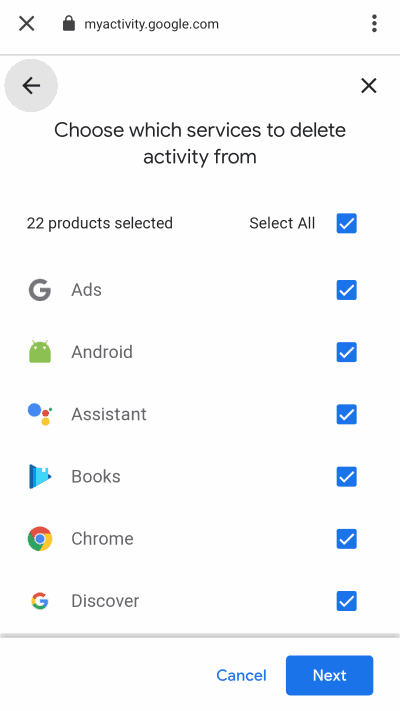The screenshot displays the interface of an Android phone accessing the "My Activity" section of Google services, specifically under the URL "myactivity.google.com." The background is white and sparse, with a light gray theme extending across various elements. 

In the top left corner, there is a gray "X" icon, followed by a padlock symbol indicating a secured page. On the top right, there are three vertically aligned dots suggesting additional menu options. A light gray line runs horizontally across the screen, with a light gray circle containing a dark gray back arrow on the left-hand side and a dark gray "X" on the right-hand side.

Below this line, the header states "Choose which services to delete activity from," hinting at an activity management function. The interface displays '22 products selected' on the left, and 'Select all' aligned to the right, next to a selected blue checkbox with a white check mark.

The selected items are illustrated with both icons and text descriptions. They include:
- A gray Google "G" with the label "Ads"
- A green Android icon labeled "Android"
- The colorful Google Assistant logo marked "Assistant"
- A blue play button icon for "Books"
- The Google Chrome icon under the label "Chrome"
- The colorful Google "G" indicating "Discover"

Separating this section is a thicker light gray line. At the bottom, blue text labeled "Cancel" appears on the left, and a blue button with white text that reads "Next" is situated on the right.